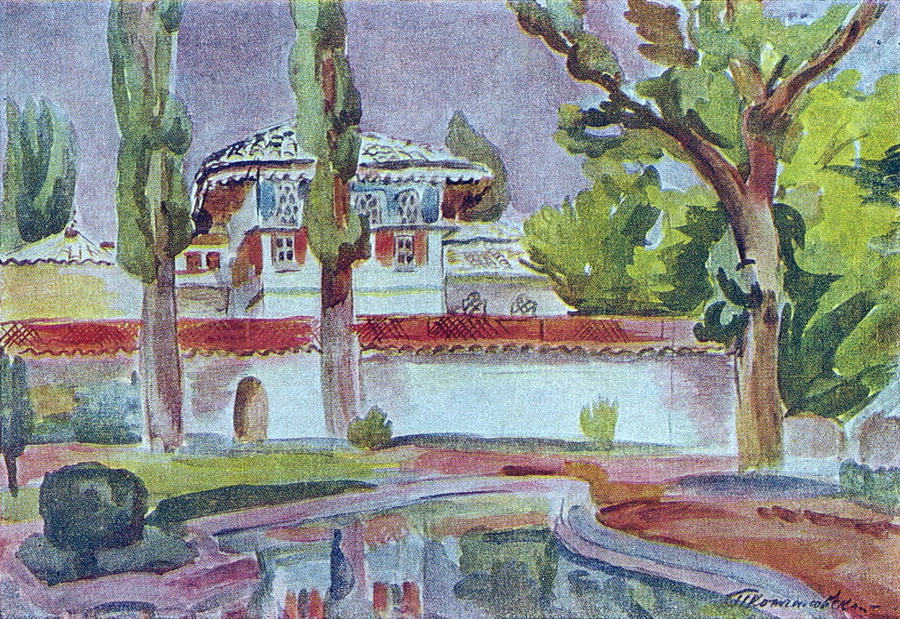This is a horizontally aligned rectangular watercolor painting depicting a colorful, two-story house with a white roof. The upper part of the house is painted blue, while the lower part is red with white accents all over. The house has red shutters on the bottom floor and blue shutters on the top floor. In front of the house is a serene, small body of water, likely a pond, capturing the reflections of a large tree situated on the right side with a brown trunk and lush green leaves. The background sky is rendered in shades of gray, adding a moody atmosphere to the scene. On the left side, one can see several bushes and green lawn areas. There are three trees in the foreground, with their reflections visible in the water below. A red fence runs above a white wall that traces across the center horizon of the image. The bottom right corner of the painting features a signature starting with a T, possibly followed by a K, although it's difficult to decipher completely. The overall composition is vibrant, with a mix of browns, greens, blues, and pinks, adding depth and richness to the scene.